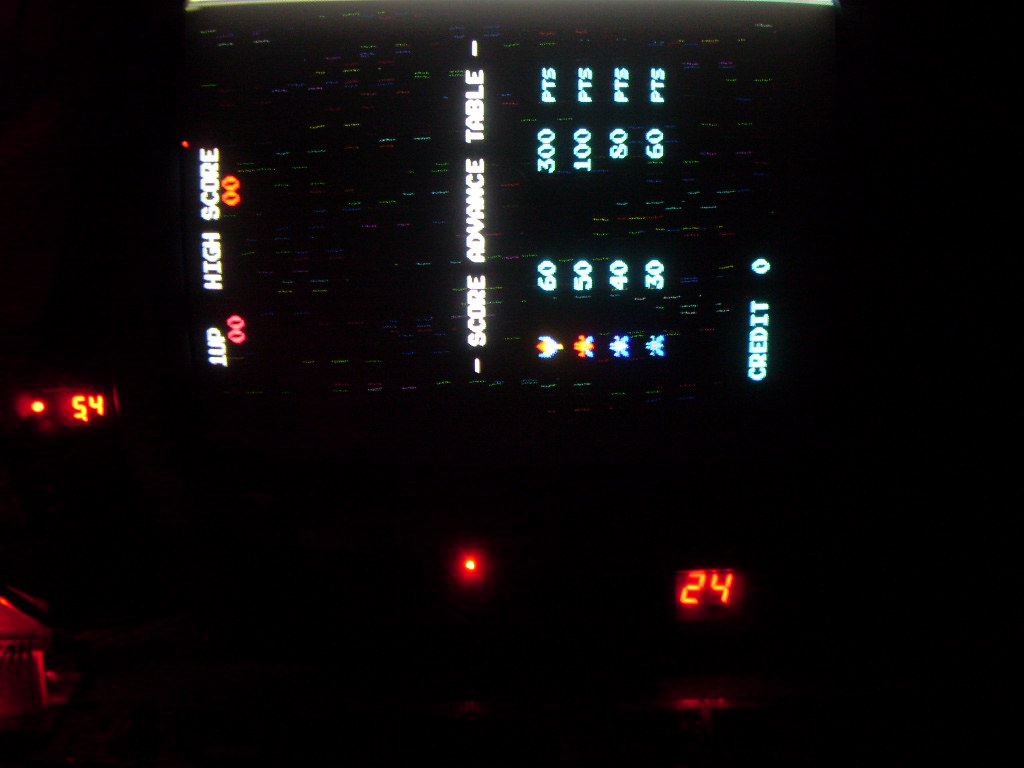The image depicts a highly contrasted, dark scene centered around an arcade screen titled sideways. The arcade screen's illuminated elements stand out vividly against the black backdrop of the room. In the middle left part of the screen, the number "54" is highlighted in orange, while the number "24," also in orange, is visible to the right of the center. The scene is partially lit by an intense red light located in the lower third central portion of the image, which contributes to the mystical atmosphere.

Reading along the horizontally turned screen, you’ll notice "One Up" indicating a single player is active, followed by "0-0 High Score" and "0-0 Score." Below this, the "Score Advance Table" is displayed prominently, listing high scores: 300 points for a score of 60, 100 points for 50, 80 points for 40, and 60 points for 30. Further down, the screen informs there are no credits remaining, marked by "0 Credits".

The enigmatic quality of the image, coupled with the tilted screen, orange highlights, and a grid laid on its side, gives a surreal and disorienting effect, drawing the viewer into the nostalgia of classic arcade gaming.